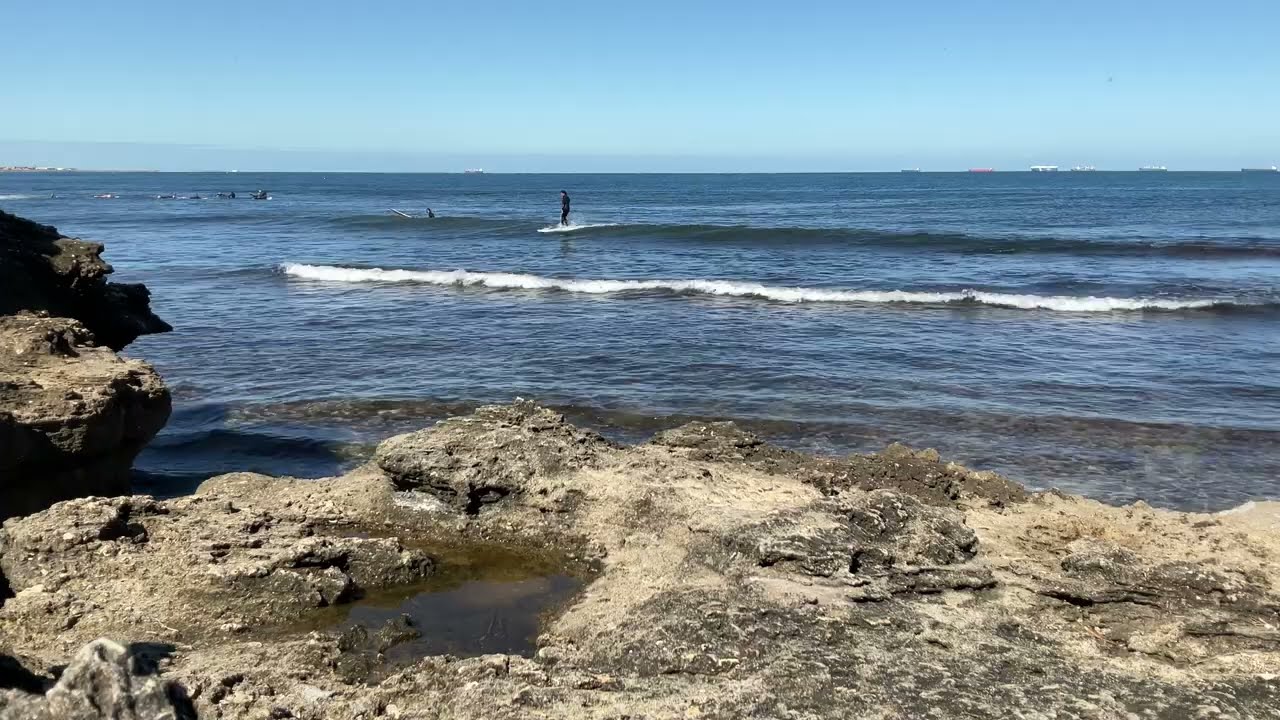The horizontally aligned rectangular picture captures a serene beach scene in the daytime. The foreground is characterized by a rocky, uneven terrain, with shades of tan and dark brown, and small puddles nestled among the rugged rock formations. Taller boulders rise on the left side. The middle portion of the image is dominated by a vast, clear blue ocean, showcasing gentle waves with white tips approaching the shore. Central to the photo, a surfer rides a modest two-and-a-half-foot wave, while another surfer to his left has his surfboard protruding from the water. In the far distance on the left, indistinguishable objects that could be people or boats dot the horizon. The clear blue sky above the ocean completes the tranquil scene. On the horizon, faint outlines suggest the presence of buildings or a mountain range, adding depth to this peaceful and relaxing coastal view.